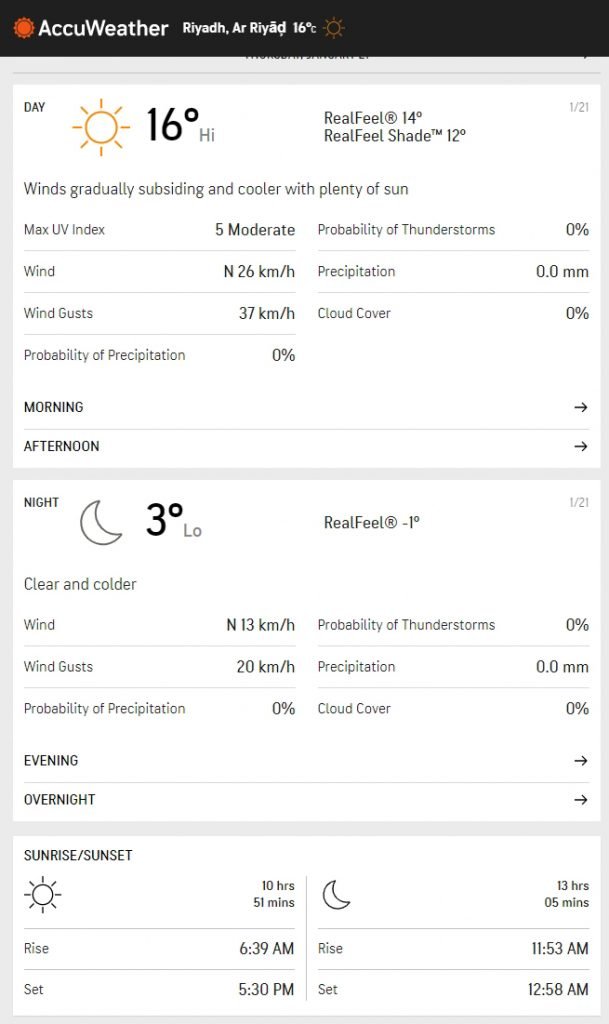The image is a detailed screenshot of the AccuWeather app interface displaying weather information. At the top, the AccuWeather logo accompanied by a sun icon is visible, indicating the app's branding. Below the logo, the location is labeled as "Rite Aid" (incorrectly spelled "R-I-E-A-D"), with a current temperature of 15 degrees Celsius.

The interface is divided into three distinct sections:

1. **Daytime Forecast:**
   - **Top Box:** Displays "Daytime" with a high of 16 degrees Celsius. The "RealFeel" temperature is noted as 14 degrees Celsius, and "RealFeel Shade" as 12 degrees Celsius.
   - **Description:** Clear skies with cooler temperatures due to subsiding gusts.
   - **Columns:**
     - Left Column: Maximum UV Index, Wind, and Dust; Probability of Precipitation.
     - Right Column: Probability of Thunderstorms, Precipitation, and Cloud Cover.
   - **Options:** Users can toggle between morning and afternoon forecasts using the arrows provided.

2. **Nighttime Forecast:**
   - **Middle Box:** Features a low of 3 degrees Celsius and a moon icon indicating nighttime. The "RealFeel" is -1 degrees Celsius.
   - **Description:** Clear and cooler conditions.
   - **Columns:**
     - Left Column: Wind, Rain, and Dust; Probability of Precipitation.
     - Right Column: Probability of Thunderstorms, Precipitation, and Cloud Cover.
   - **Options:** Users can view evening and overnight forecasts, navigable via arrows.

3. **Sunrise and Sunset Information:**
   - **Bottom Box:** Displays sun and moon icons without a temperature reading.
   - **Sunrise:** 10 hours 51 minutes of daylight, rising at 6:39 a.m.
   - **Sunset:** Noted separately to the right with 13 hours 5 minutes of nighttime, rising at 11:53 a.m. and setting at 12:58 a.m.

This detailed information offers a comprehensive look at the weather conditions and forecast options available within the AccuWeather app.